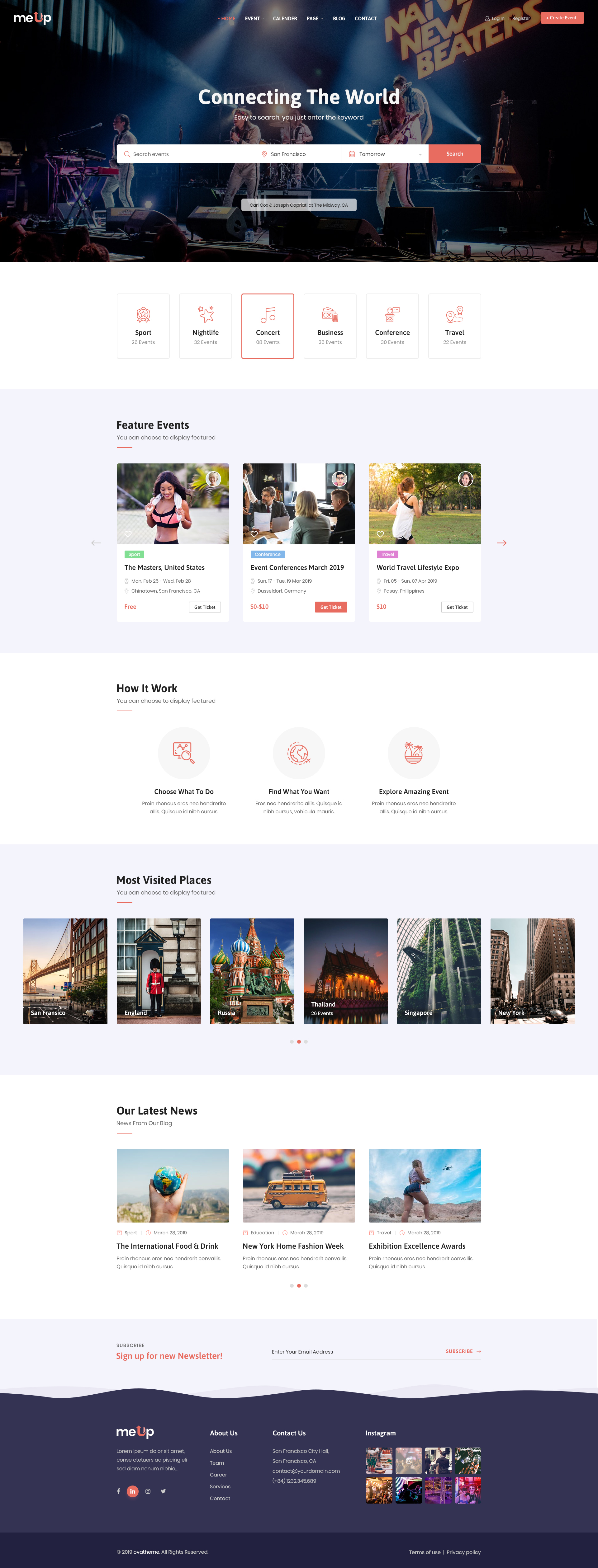The image depicts a vibrant and user-friendly website interface for an event search platform named "Me Up," with the "U" and "P" stylized as an upward arrow. The homepage features a dynamic screenshot of a band performing live, accompanied by the slogan "Connecting the World." Users are guided to search for events by entering relevant keywords in designated search bars for location, time, and category.

At the forefront is an intuitive search section, allowing users to filter events based on various categories, including Sports, Nightlife, Concerts, Business, Conferences, and Travel. Below the search functionality, there is a section showcasing featured events. It displays detailed information about each event, including the name, brief details, ticket prices, and a button to purchase tickets.

Further down, the "How It Works" section provides a clear, step-by-step guide on utilizing the platform to find and explore events. Following this, a "Most Visited Places" section presents a visually appealing array of banner images featuring popular destinations such as San Francisco, England, Russia, Thailand, Singapore, and New York.

The "Latest News" section highlights the platform's blog with three side-by-side articles, each accompanied by an image. Towards the bottom of the page, users are invited to sign up for a newsletter and can find additional details about the platform, including contact information and a link to their Instagram page.